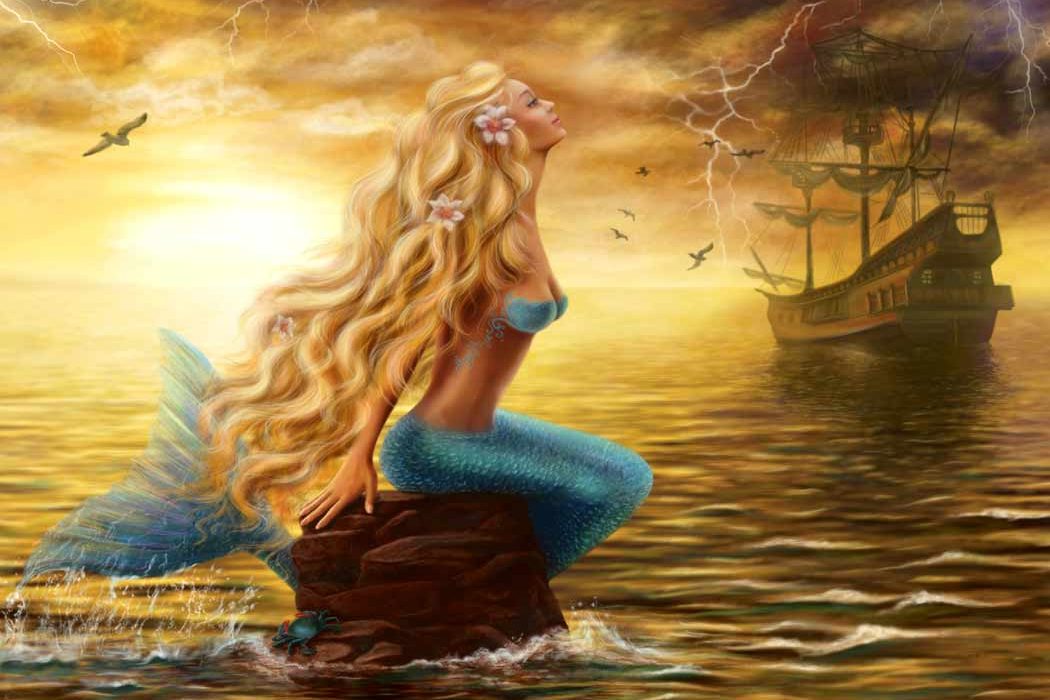The image is a digital creation or painting capturing a moody seaside scene during sunset. The sky, bathed in a golden-orange hue, is contrasted by dark, stormy clouds pierced by jagged lightning bolts. In the background, seagulls glide through the air, and an old pirate ship with its sails secured to the masts floats on the right side of the frame.

Dominating the left side, a rock juts out of the water with a blue crab perched on its ledge. Atop the rock sits a mermaid with long, flowing blonde curls adorned with three white and pink flowers. She wears a blue bra and her shimmering blue tail extends behind her, with its fin visible splashing in the water. Her posture, with arms and hair cast back, gives her a majestic yet wistful presence.

The tranquil yet dramatic interplay of light, color, and elements adds depth to this evocative maritime scene, blending kitschy charm with a touch of fantasy.